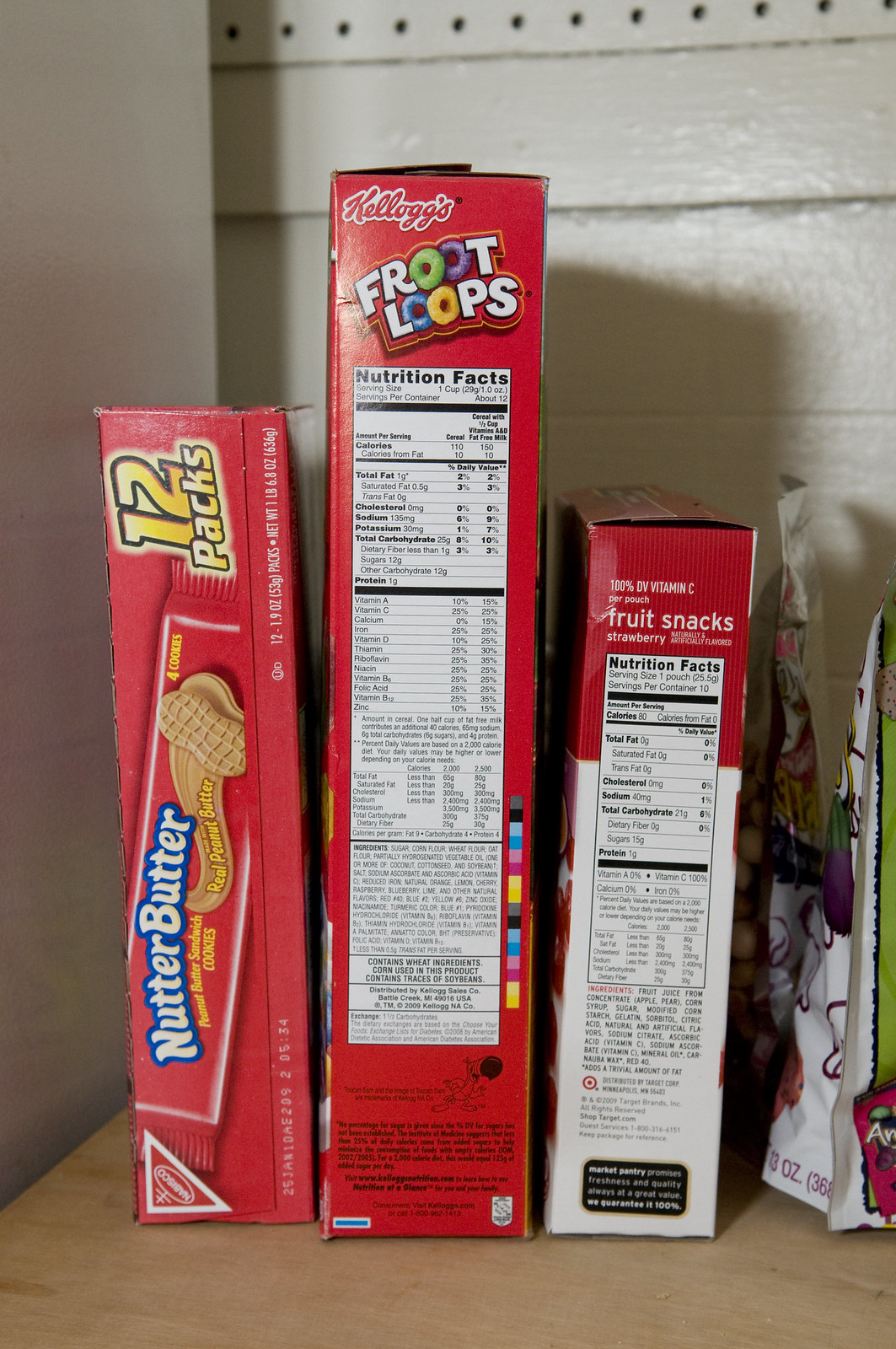Close-up of a trio of food boxes neatly arranged on a light-colored wooden shelf against a white-painted wooden wall. Each box is a vibrant shade of red. On the left, a multi-pack box of Nutter Butter single-serve packs of cookies stands vertically on its side. The Nabisco logo is prominently displayed at the lower-left corner of the box, which would be the top left if positioned horizontally. The Nutter Butter cookie package is illustrated diagonally through the center, with a bold "12 packs" label in yellow at the top-right corner of the box (appearing at the bottom in this vertical orientation).

The middle box features a side view of a Froot Loops cereal box, displaying the comprehensive Nutrition Facts panel. The iconic Kellogg's logo is situated in the top left corner, with the Froot Loops branding angled centrally. The long, rectangular white Nutrition Facts panel occupies much of the visible surface.

To the right sits a vertically standing box labeled "Fruit Snacks" in modest lettering, with "Strawberry" inscribed in smaller type below. This side also showcases the Nutrition Facts panel.

Adjacent to the food boxes, a small aluminum bag, presumably containing dog treats, lies ripped open in the center. Peeking into the scene from the left, a white metal edge suggests the presence of a refrigerator. The entire setup rests against a white-painted wooden backdrop, creating a crisp, organized visual.